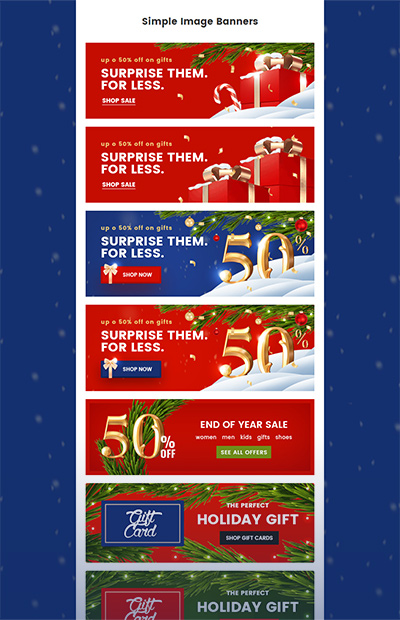The image depicts a vertical screenshot from a mobile-designed website, likely intended for web developers or graphic designers. It showcases eight distinct image banner designs, all sharing the same core message but featuring various visual elements. Each banner includes a "Shop Now" button, with some styled simply and others creatively shaped like presents. 

The designs vary in imagery, with several banners adorned with festive elements such as trees, gifts, and snowbanks. Some banners highlight a bold "50% Off" message, prominently displayed in eye-catching gold text. In one design, the discount message is superimposed over what seems to be a branch or a wreath. Other designs feature illuminated trees either at the top, bottom, or both, set against diverse background colors.

Overall, while the central information remains constant, the background images, colors, and decorative elements differ across the banners, offering a variety of stylistic options for different visual preferences.